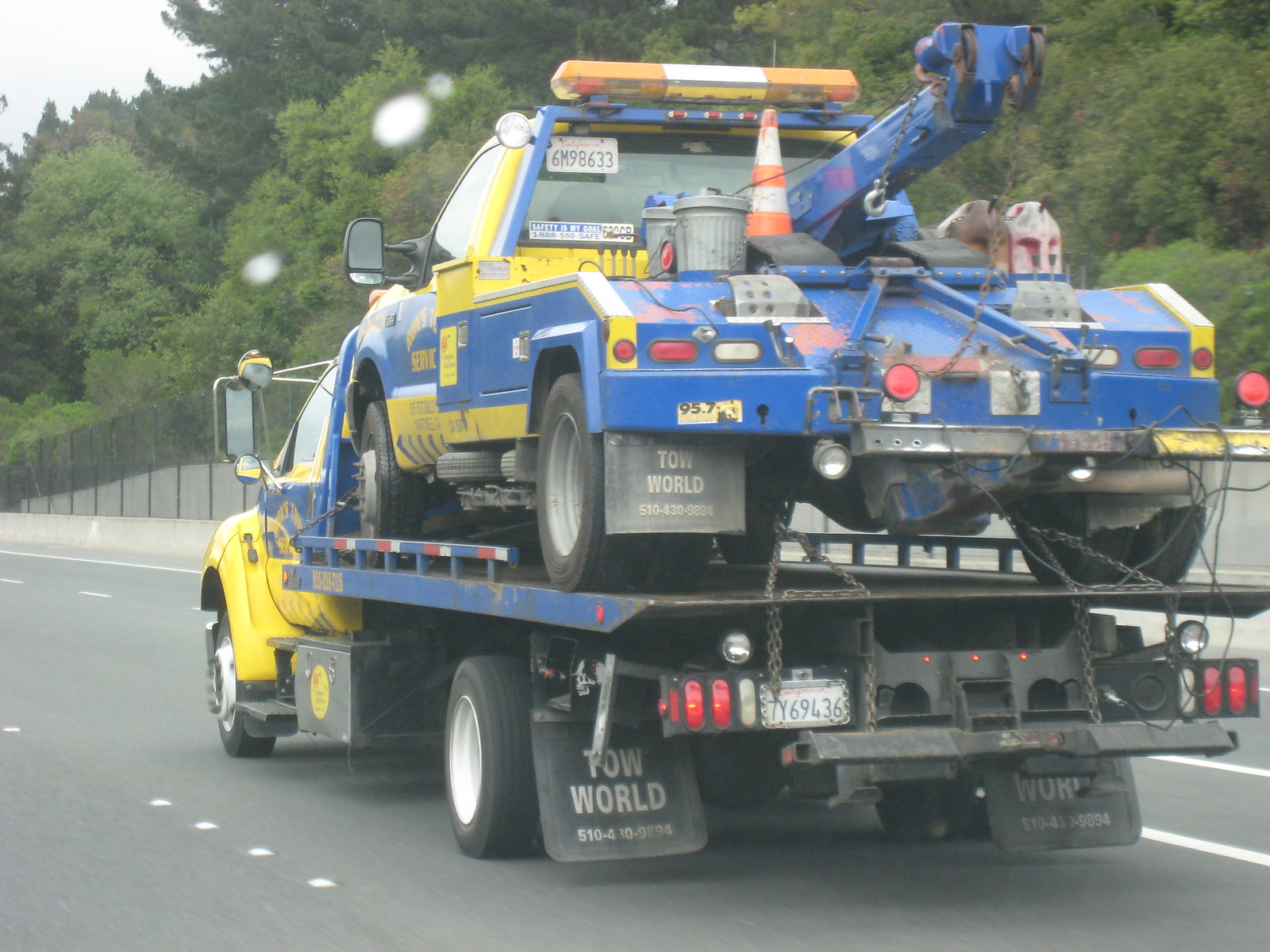This photograph captures a humorous scene of a blue and yellow flatbed tow truck from the company Tow World hauling another tow truck of the same colors and company. The flatbed tow truck, which winches vehicles onto its flatbed, is transporting a second tow truck designed with a boom and winch to lift cars. Both vehicles feature mud flaps bearing the Tow World logo. The secondary tow truck on the flatbed carries metal garbage cans and an orange traffic cone, and displays two red lights with a gold section between them on top. They are traveling on an interstate or multi-lane highway, bordered by a fence and barrier on the right side. Behind the fence stretches an embankment rich with greenery, abundant trees, and foliage, against a light-colored sky, adding natural beauty to the otherwise comical and peculiar scene.